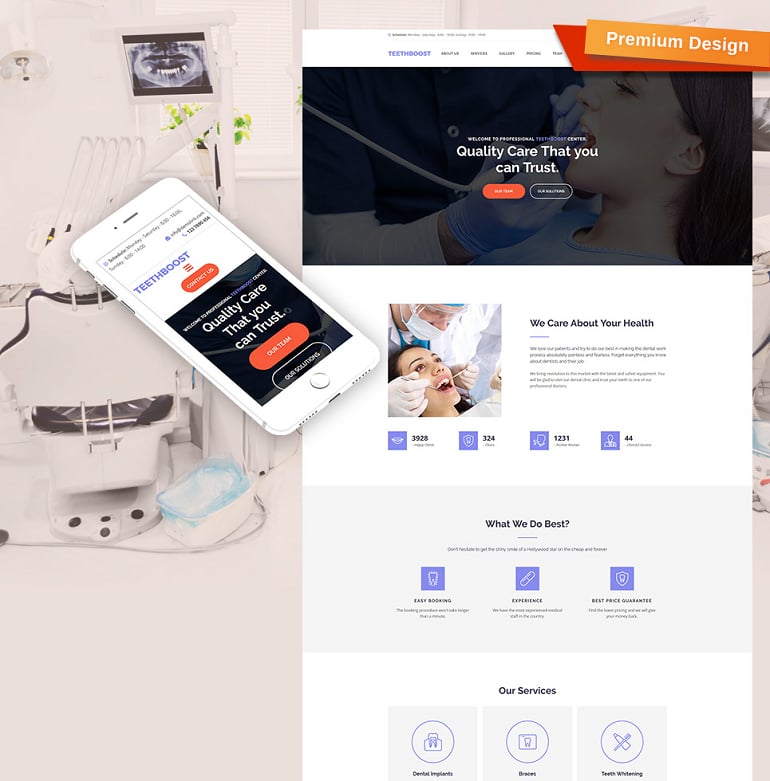This image is a comprehensive mock-up of a dental care website homepage, accompanied by a digitally created smartphone overlay. Here is a detailed description of the elements within the image:

**Webpage Layout:**

- **Right-Hand Section:**
  - Features a dental hygienist or dentist, identifiable by their attire, working on a patient's teeth. 
  - The patient, a light-skinned woman with shoulder-length brown hair, is receiving dental care.
  - The dental professional is dressed in purple gloves, a long-sleeved white T-shirt, and a dark blue dress shirt.
  - Prominent text overlays include "Welcome to Professional," followed by "Teeth Something Center" in bold white text with the "Teeth Something" portion highlighted in purple.
  - Larger white bold text reads, "Quality Care That You Can Trust."
  - Three clickable buttons are displayed: one orange, another bordered in white with white text, and one more unspecified.

- **Top Left Corner:**
  - The branding "Teeth Boost" appears in purple.

- **Additional Overlays (Right-Hand Side):**
  - Two rectangular shapes: one dark red, the other orange with white text stating "Premium Design."

**Smartphone Interface:**

- The smartphone screen shown over the webpage presents a clean, white background with black text at the top for time and location.
  - The title "Teeth Boost" is reiterated in purple.
  - An orange-red settings icon with three lines is also present.
  - An orange "Contact Us" button with bold white text.

- **Further Details:**
  - A black section with white text repeating "Welcome to Professional's Teeth Boost Center," again highlighting "Teeth Boost" in purple.
  - The slogan "Quality Care That You Can Trust" in large, bold white text.
  - An orange circle with bold white text inside that reads, "Our Team."
  - An oval bordered in white with an unspecified text concerning "Followers."

**Additional Elements:**

- A dental light and an X-ray are visible on the left-hand side.
- Another scene depicts a woman, smiling with pink lips and shoulder-length brown hair, receiving dental care from a dentist in blue scrubs and a white mask, parting her mouth.
  - A message "We Care About Your Health" is in bold black text, but the surrounding text is too small to decipher.

**Statistical Data:**

- Numeric data in purple squares:
  - 3,928 next to a smiley logo.
  - 3,024 next to a shield.
  - 1,231 next to a person yelling.
  - 44 next to a silhouette of a person standing.

- "What We Do Best" in bold black, followed by indistinct smaller text.

**Service Features:**

- Represented by colored icons and text:
  - A tooth in purple stating "Easy Booking" in bold black.
  - A pill-like silhouette inside a purple square indicating "Experience" in bold black.
  - A shield with a tooth drawn in white within a purple square, labeled "Best Price Guarantee."

**Services Offered:**

- Text "Our Services" in bold black at the bottom.
  - Dental Implants: illustrated with a purple circle featuring a tooth and gum line.
  - Braces: shown with another tooth icon within a purple square and circle.
  - Teeth Whitening: depicted with a piece of toothpaste and a toothbrush in purple within a worded circle.